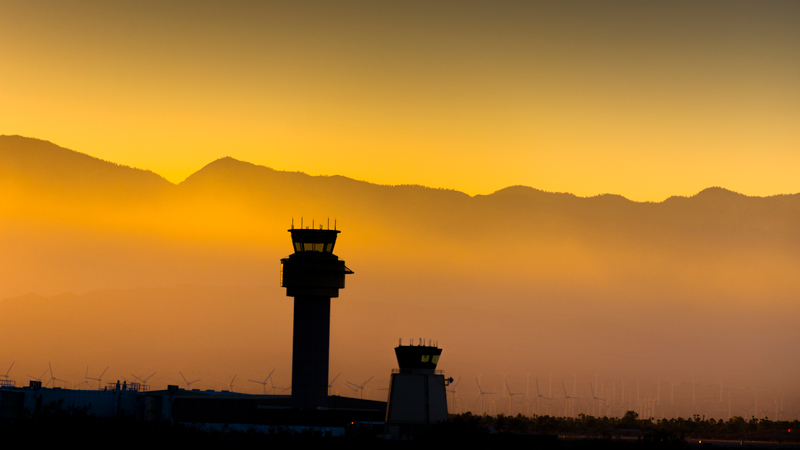This photo, likely taken at sunset given the yellow glow on the horizon, captures two towers positioned in shadow. The taller tower on the left looms over the shorter tower on the right. In the distant background, partially shrouded by fog or clouds, a wind farm with several large, three-bladed wind turbines can be seen. Mountains border the horizon, appearing dark against the fading light. Despite the initial ambiguity regarding the towers' functions, they resemble watchtowers, possibly for a prison or an airstrip. The bottom part of the image remains dark, with no visible buildings or fencing, though the turbines add a distinctive feature to the landscape.